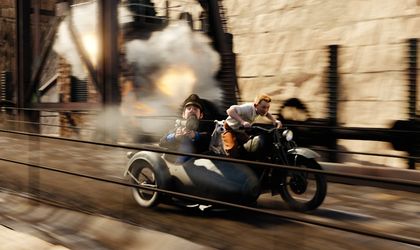The image features a dynamic scene with a motorcyclist speeding through an alleyway on a sleek, black and chrome motorcycle. The motorcyclist, wearing a white t-shirt and brown pants, is intensely focused, leaning over the handlebars as he races alongside a building. Attached to the motorcycle is a sidecar where a secondary figure sits – a man with a hat and a mustache, wearing a blue-black uniform and holding a package. A white dog can be seen perched behind the motorcyclist. Smoke billows behind them, suggesting a fast getaway, while in the background, there is a fence and what appears to be a brown house engulfed in flames or an explosion. The chaotic and almost cartoonish energy of the scene is heightened by the detailed depiction of the characters and their surroundings.